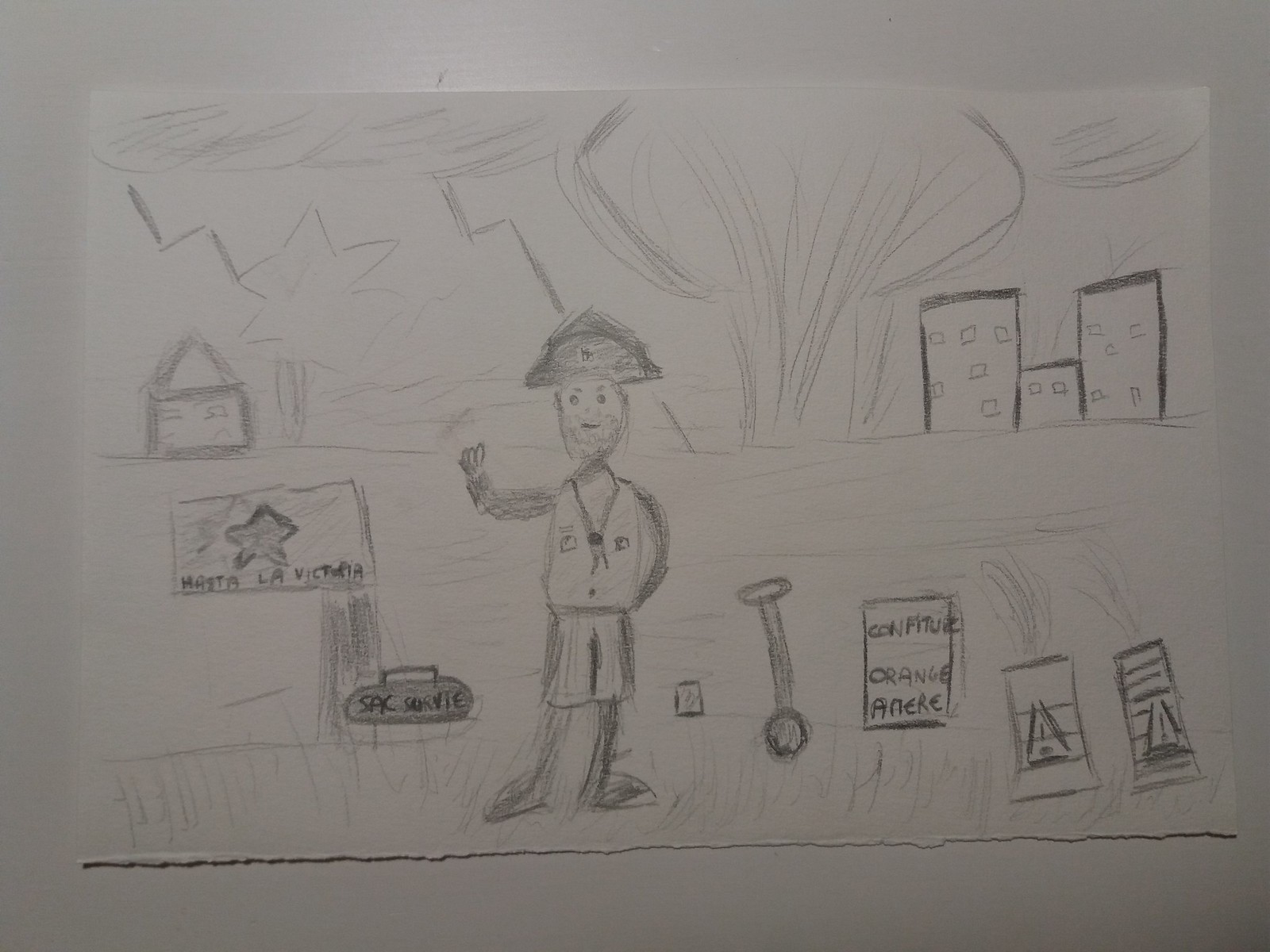This detailed pencil sketch, rendered entirely in black and white, is drawn on a white sheet of paper placed on a similarly light-colored surface. 

The focal point of the image is a human figure standing prominently in the foreground. The figure is depicted with a friendly demeanor, characterized by their right hand raised in a welcoming gesture. Their left arm is bent behind their back, with the hand curving around the midsection. The figure is adorned with a hat resembling that of a fireman, intricately shaded with pencil. Facial features, including the eyes, nose, and mouth, are clearly rendered.

The attire of the figure consists of a vest, evident from the buttons drawn on the upper part of the clothing, and shorts. Adjacent to the figure is a radio or similar equipment, possibly a bag, labeled with the letters "S-A-C-S-U-R-B-I." The sketch also includes the words "Hasta la victoria, confitur orange," suggesting a possible message or theme, although the specific language remains unclear.

In the background, various structures such as buildings and houses are faintly outlined. The sky above these buildings seems to depict an explosion or potentially abstracted tree forms, contributing to a sense of depth and narrative within the artwork. The entire composition showcases the artist's skill in pencil shading and provides a rich, detailed visual story.